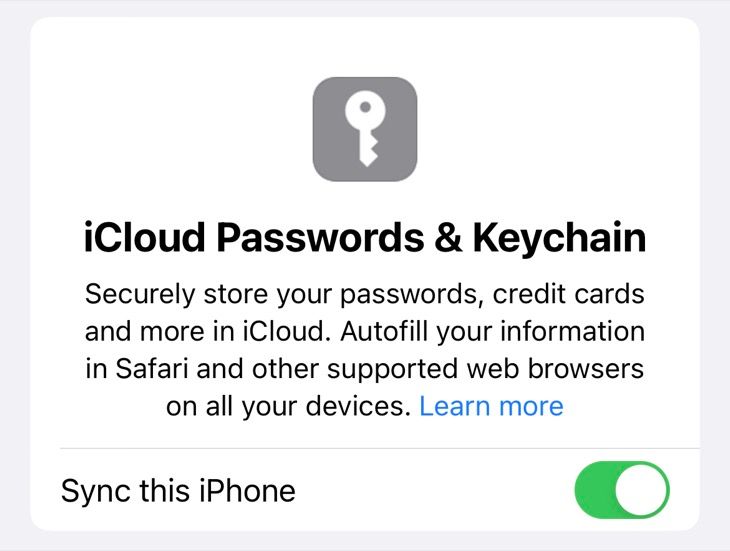### Detailed Caption for the Screenshot of iCloud Passwords and Keychain Settings on an iPhone

This image is a screenshot from an iPhone displaying the settings for iCloud Passwords & Keychain. At the top of the screen, there is a key icon which likely represents security or the keychain feature. Directly below the icon, the heading "iCloud Passwords & Keychain" is prominently displayed in bold text.

The section is designed to securely store your passwords, credit cards, and other sensitive information in iCloud, allowing for seamless auto-fill of your information in Safari and other supported web browsers across all your devices. Below the heading, there is a description written in smaller, non-bold black text that elaborates on these features.

A notable feature is the "Sync this iPhone" toggle switch, which is turned on. The switch is positioned to the right and is green, indicating that synchronization for this iPhone is currently enabled. This toggle is clearly visible and easily accessible, allowing users to quickly enable or disable this feature.

Additionally, there is a blue hyperlink labeled "Learn More" embedded within the text, which, when clicked, provides further information about the iCloud Passwords & Keychain settings.

The interface is straightforward, providing clear and concise information relevant to passwords and keychain management, making it easy for users to understand and navigate the settings.